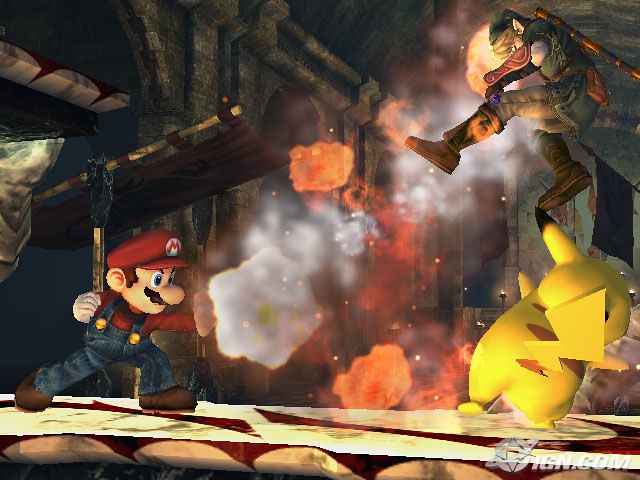The image is a detailed screenshot from a video game, featuring well-known Nintendo characters in a dynamic scene. At the bottom left, Mario, donned in his iconic red hat with a white circle and "M," is throwing a fireball, which has struck another player, sending them flying through the air. The action takes place on a raised red and white platform, resembling a bridge. 

Further along the platform, Pikachu, characterized by its yellow body and lightning bolt-shaped tail with black-tipped ears, is standing steadfast. Above Pikachu, Link from the Zelda franchise, identifiable by his blonde hair, elf ears, and green tunic and hat, is caught mid-air in a leap. 

The background sets a dramatic tone with its castle-like architecture and seems to depict the interior of a building. Red hues dominate the scene, highlighted by flowing lava and emanating smoke, suggesting a dangerous environment. The entire image is free of text except for a watermark in the bottom right corner that reads "IGN.com," solidifying its origin as a video game screenshot.